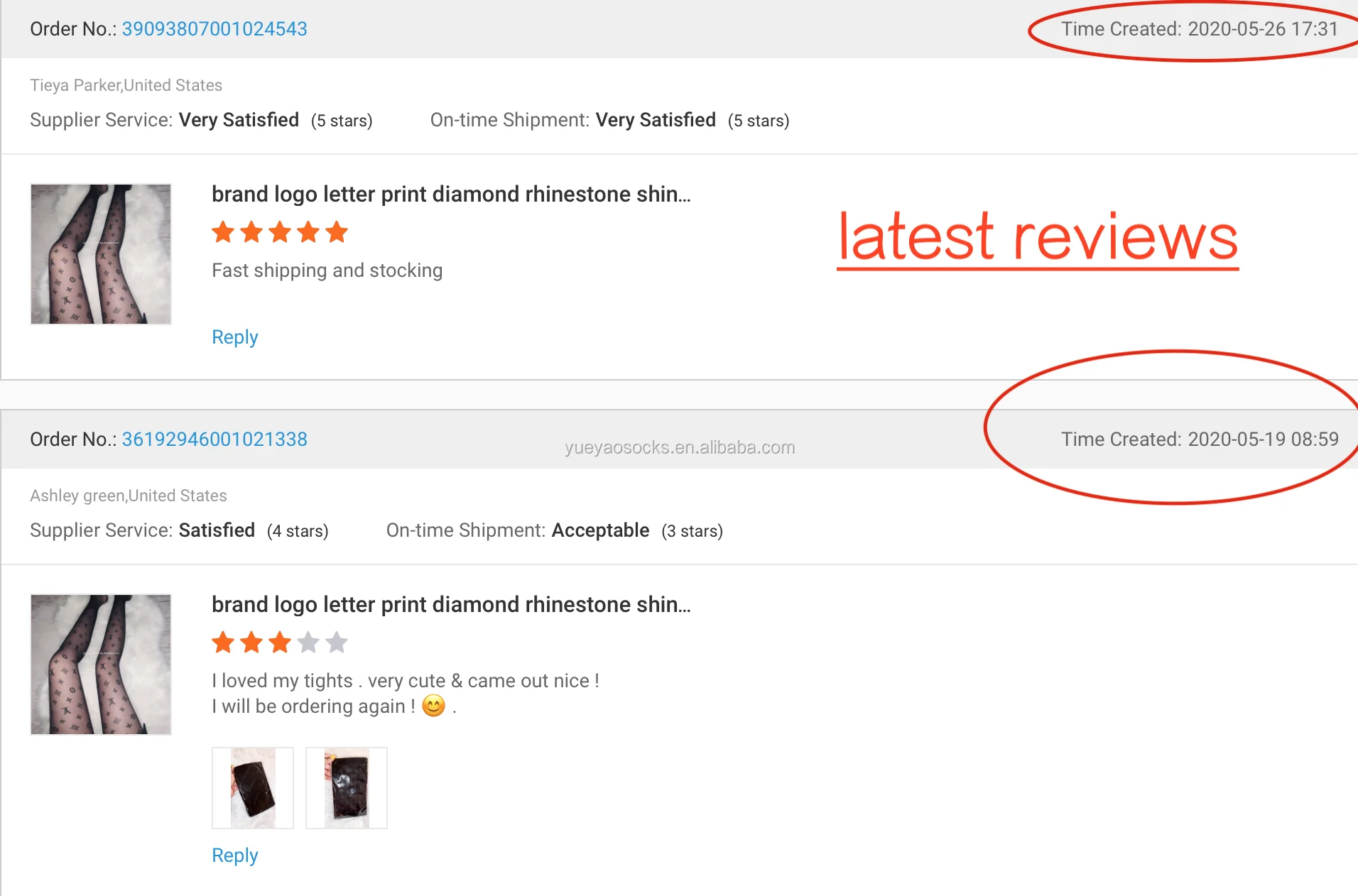These are two side-by-side, detailed images of order confirmations and reviews from an online shopping platform. 

**Left Image:**
At the top of the image, the order number "3909-380-700-1024543" is prominently displayed. The seller is identified as "Tierpark, United States" in a light gray font. There are satisfaction ratings listed:
- **Supplier Service:** Very satisfied (5 stars)
- **On-time Shipment:** Very satisfied (5 stars)

In the upper right corner, in a gray font, the timestamp "2020-05-26 17:31" is displayed, highlighted by a red border.

In the main body, there's a picture featuring a woman's legs adorned with sleek, dark stockings decorated with small diamond-like images. The product description reads: "Brand logo, print diamond, rhinestone", rated five stars, with comments highlighting "Fast shipping and stockings."

**Right Image:**
This image mirrors the structure of the first but with different details. The order number here is "3619-946-0012-1338." It also features the URL "YEYAOSOCKS.EN.Alibaba.com," indicating a Chinese online store. The order timestamp shows "2020-05-19 08:59."

Listed below this are the customer details: "Ashley Green, United States." The ratings are slightly lower:
- **Supplier Service:** Satisfied (4 stars)
- **On-time Shipment:** Accepted (3 stars)

The image below contains the same stockings with a woman's legs and reads: "Brand logo, letter print diamond, rhinestone," but this time with a three-star rating. A customer review says, "I love my tights. Very cute and came out nice. I'll be ordering again."

At the bottom of both images are a series of small icons, including what appears to be representations of a phone and potentially an iPad, though the details are faint. Each section concludes with a blue "Reply" button.

Together, these images provide a contrasting yet comprehensive overview of two different customer order experiences from the same seller, highlighting product satisfaction and delivery efficiency.